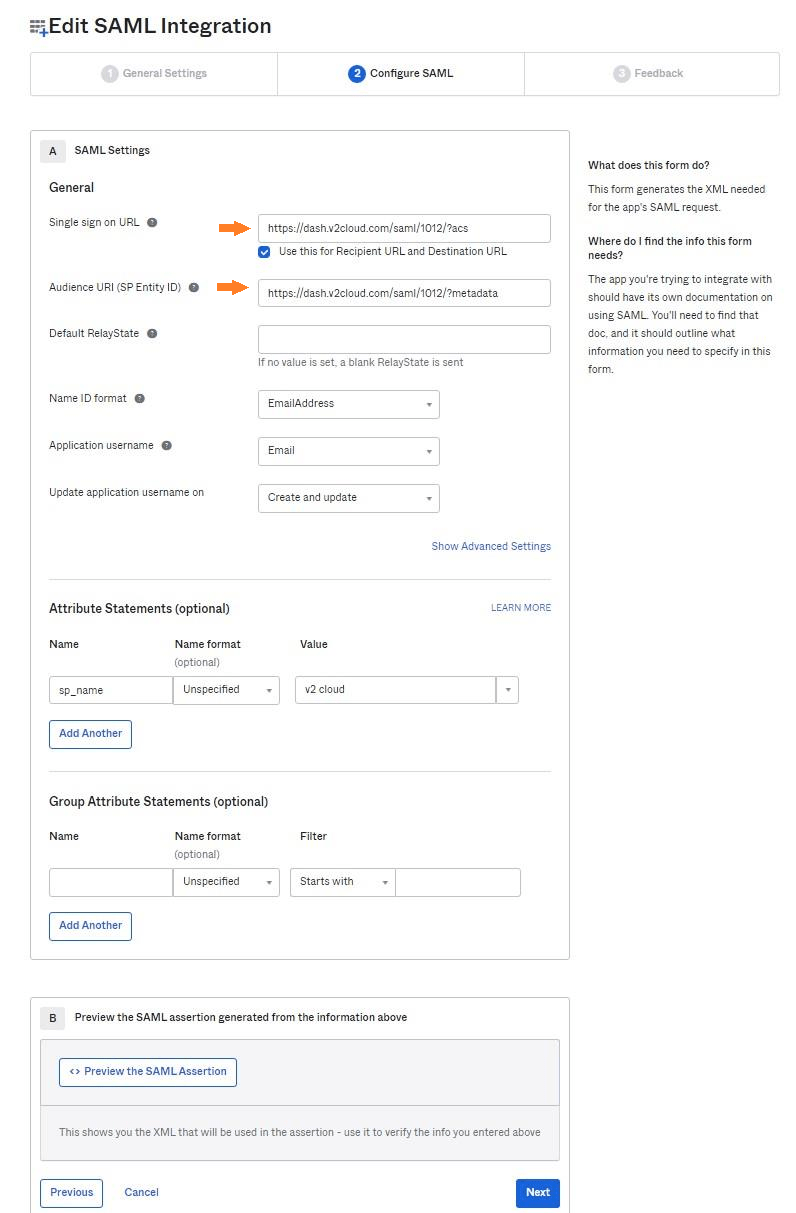This image depicts a detailed view of a settings landing page for editing SAML integration. At the top, the title "Edit SAML Integration" is prominently displayed. Below the title, there is a navigation bar with options such as "General Settings," "Configure SAML," and "Feedback." The current selection is the "Configure SAML" section, which is highlighted.

In this "Configure SAML" section, the first item is labeled "SAML Settings," which is prefixed by a letter "A". This section includes fields for "General Single Sign-On URL," "Audience URL," "Default Relay State," "NameID Format," and "Application Username." Additionally, there is an option to "Update Application Username."

At the bottom right corner, there is a button labeled "Next." To the right side of the form, an explanatory note reads, "This form generates the XML needed for the app's SAML request," providing context for the purpose of the settings.

The image also includes arrows pointing specifically at the "Single Sign-On URL" box and the "Audience URL" box, indicating these are points of interest or necessary input fields in the configuration process.